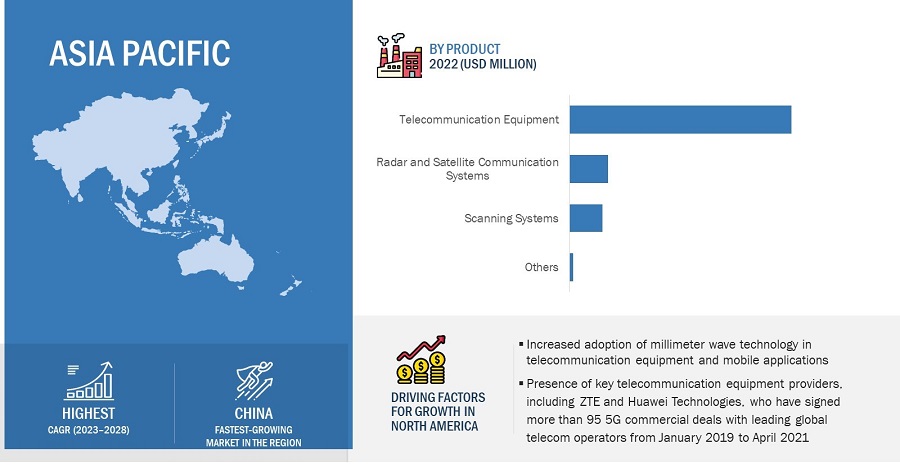The image is an analytical business infographic, displaying detailed information about the Asia-Pacific region and the telecommunications market. The left side features a blue and white map of Asia-Pacific, highlighting countries such as China, Russia, India, the Philippines, and Vietnam. Below the map, the graphic notes that China is the fastest growing market in the region, with an icon of a superhero emphasizing this point. It also mentions the highest CAGR (Compound Annual Growth Rate) from 2023 to 2028.

On the right side, a comprehensive horizontal bar graph presents the sales data for telecommunication equipment in the United States for 2022, measured in USD million. The graph shows telecommunication equipment as the highest category, followed by radar and satellite communication systems, scanning systems, and others. Additional graphics illustrate the driving factors for growth in North America, including increased adoption of millimeter-wave technology and significant contributions from key telecommunication providers like ZTE and Huawei Technologies.